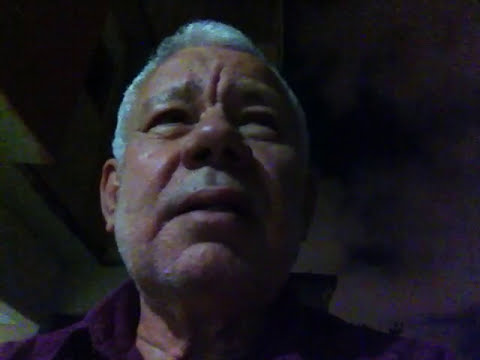This image is a close-up photograph of a man, likely in his late 50s or early 60s, looking slightly upwards from a 45-degree angle, giving a view up to his nostrils. He has short, grayish-white hair, a darker complexion, and a stubble-covered chin. He is wearing a purple or blue collared shirt, visible from his shoulders to the top of his head. His expression is neutral with his mouth closed, and he isn't directly engaging with the camera as if he might be in a video call or FaceTime session. The lighting is dim, with noticeable glare on the left side of his face, leaving the right side in shadows. The background is blurry and dark; on the left side, there's a geometric, brownish-yellow object, while the right side appears to have hazy, cloud-like material against a darker backdrop. The overall image is grainy and slightly blurry, contributing to an unclear understanding of the detailed background elements.